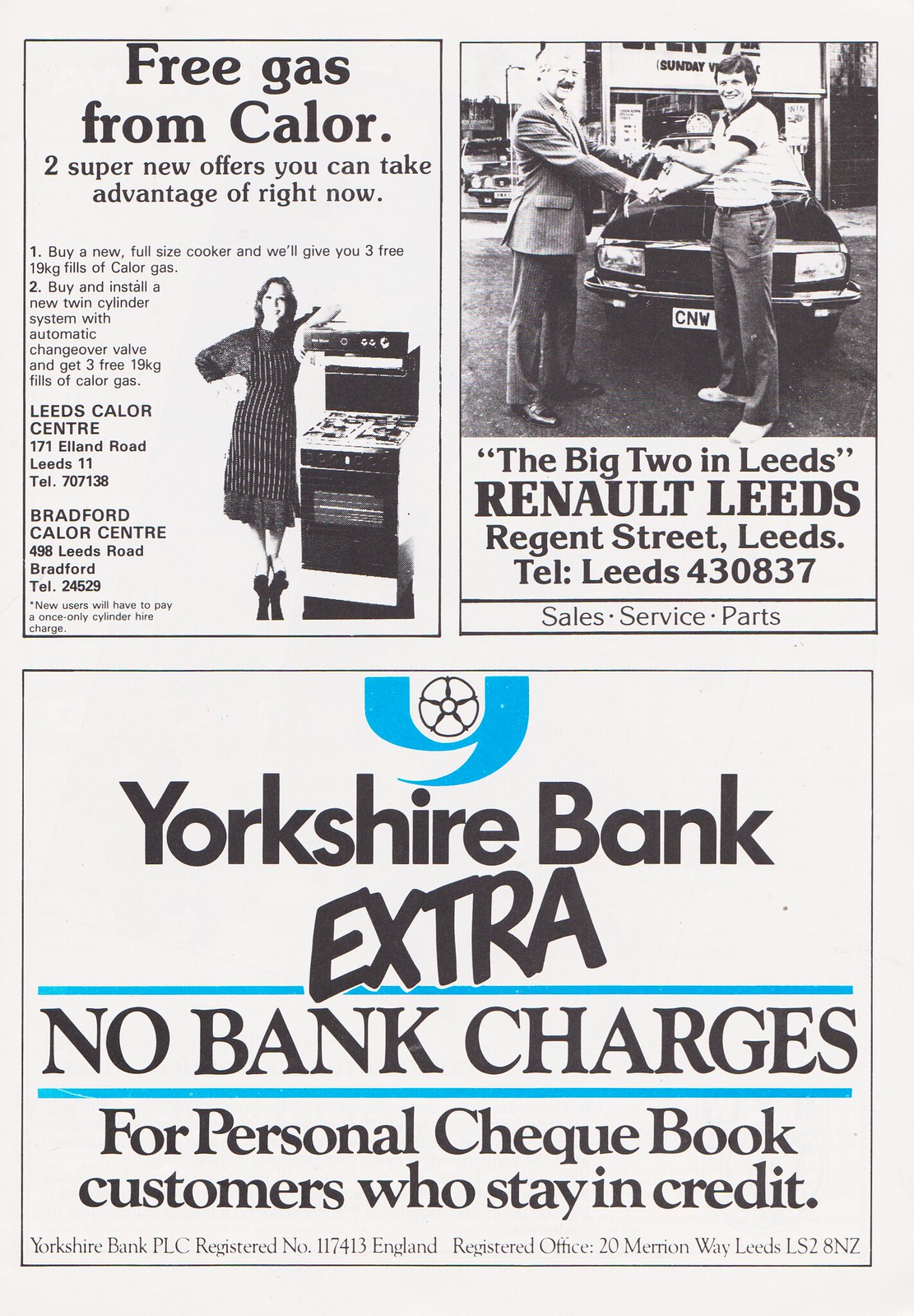This image is an old, rectangular flyer with a white background featuring three square sections—two at the top and one large one at the bottom. The flyer primarily uses black ink, with a touch of blue in the lower section.

In the top left section, there is a black and white photograph of a woman in a long black dress standing next to a gas stove. The text above her reads, "Free gas from Kohler." It further promotes "Two super new offers you can take advantage of right now." Details beneath the title mention that customers can receive free gas with the purchase of specific gas systems from Leeds and Bedford Kohler Centers.

The top right section displays a black and white image of two men shaking hands in front of a car, likely at a dealership. The accompanying text says, "The Big 2 in Leeds," followed by "Renault Leeds, Regent Street, Leeds. Telephone Leeds 430837," and also lists "Sales Service Parts."

The bottom section prominently features a logo with a black star in the center of a circle surrounded by a large blue 'Y.' The text within this section states, "Yorkshire Bank Extra," and highlights an offer: "No bank charges for personal checkbook customers who stay in credit." Additional details provide the bank's registration information and address: "Yorkshire Bank PLC, Registered number 117413, England. Registered office 20 Marion Way, Leeds. LS2 8NZ."